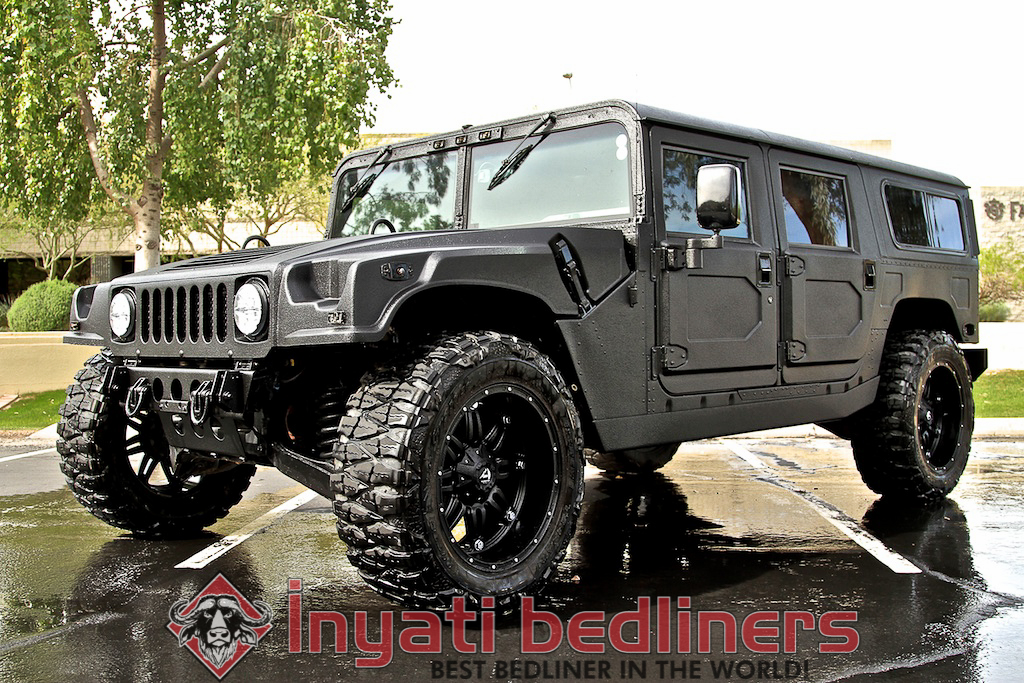This photograph features a rugged, army-grade jeep-like vehicle parked diagonally in the middle of a wet parking lot. The vehicle captures most of the image, showcasing its matte metallic silver color, flat top, and large rectangular shape. It has two doors visible on the side facing the camera, large black handles, and an elevated suspension system supporting massive tires with black rims. The headlights are circular, and the windshield wipers are prominently placed on top of the windshield.

Above the vehicle, the sky appears white, contrasting with the tree with green leaves and multiple indistinct buildings in the background, suggesting a potentially cloudy or overcast day. The ground is wet, indicating recent rainfall.

At the bottom of the image, in red text, is a watermark that reads "Iñáti Bedliners, Best Bedliner in the World," accompanied by an exclamation mark. To the left of this text is a four-sided logo with a red background featuring a water buffalo with black fur. This logo emphasizes the brand of the bedliner used in the vehicle, suggesting superior quality and toughness, complementing the vehicle's robust military aesthetics.